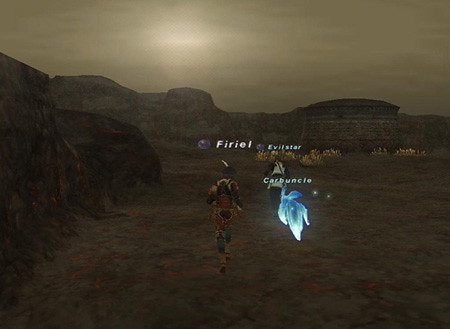This image is a dimly lit screenshot from a video game set in a vast, desolate desert landscape. The ground is a mix of browns, tans, and oranges, covered in dust with no visible green vegetation or trees. Large rocky hills and cliffs dominate the left side of the scene, while there is a large stone-like formation on the right. The sky is a gradient of light and dark gray with a small amount of sunlight piercing through the clouds at the top.

In the foreground, three characters are distinctly visible, each identified by names in white writing. "F-I-R-I-E-L" hovers above a humanoid figure dressed in full gear with yellow and red accents on their legs, stomach, arms, and head. Next to this character, "C-A-R-B-U-N-C-L-E" floats above a glowing, bluish-white, fox-like entity, adding an ethereal touch. To the right and slightly in the background, the name "E-V-I-L-S-T-A-R" appears with purple dots beside it, situated above another humanoid shape. The scene is dark and somewhat blurry, evoking a mysterious and eerie atmosphere typical of dynamic, immersive gameplay.